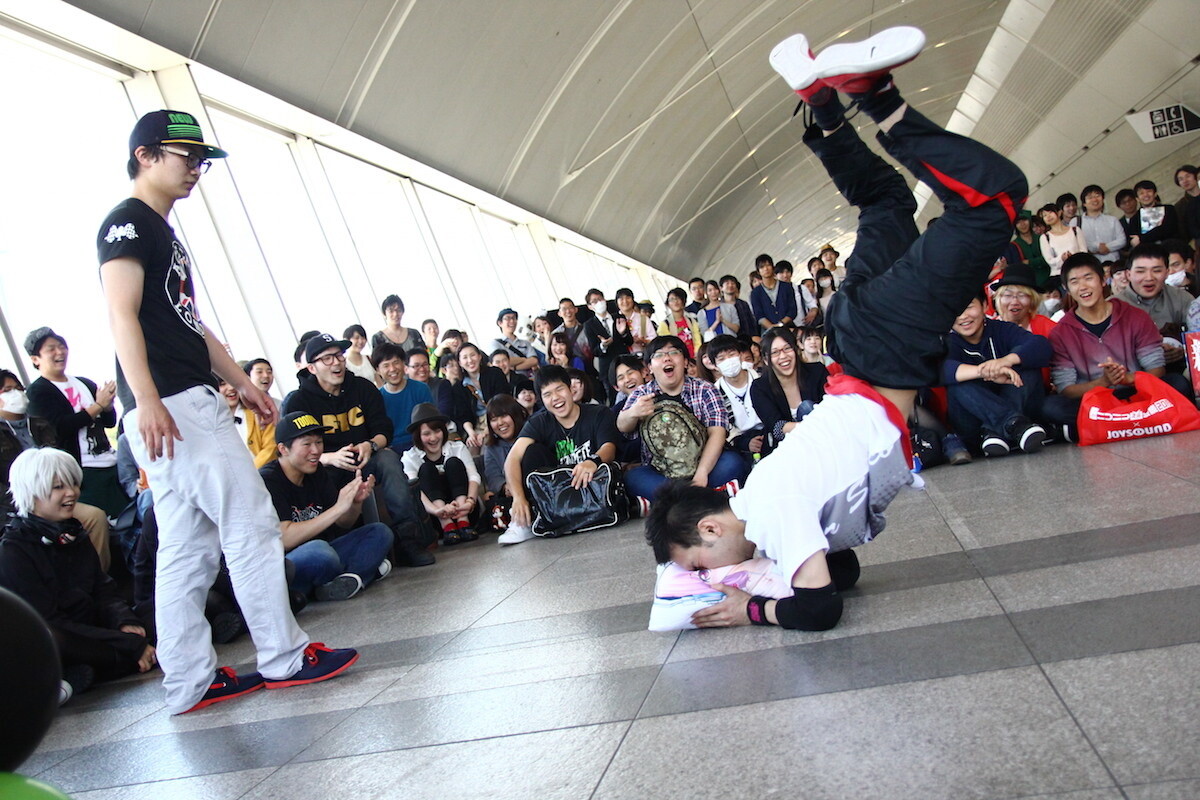In this vibrant image set in a spacious public area resembling an airport or convention center, a large crowd of over 50 people, predominantly Asian, is gathered, watching intently as a young man performs a breakdance stunt. The dancer, dressed in a white shirt, navy blue track pants, and white-red shoes with his head down into a pink and blue object, commands the center of attention. The tiles on the gray floor reflect the dynamic energy of the scene. Close by, another young man in a black shirt, cream-colored pants, navy blue shoes with red soles and laces, and a black-green cap observes the performance. The crowd, a mix of individuals donning various hats, glasses, wigs, and colorful attire including black, white, green, red, gray, yellow, and blue, adds to the lively atmosphere, with some people masked amid the assembly.